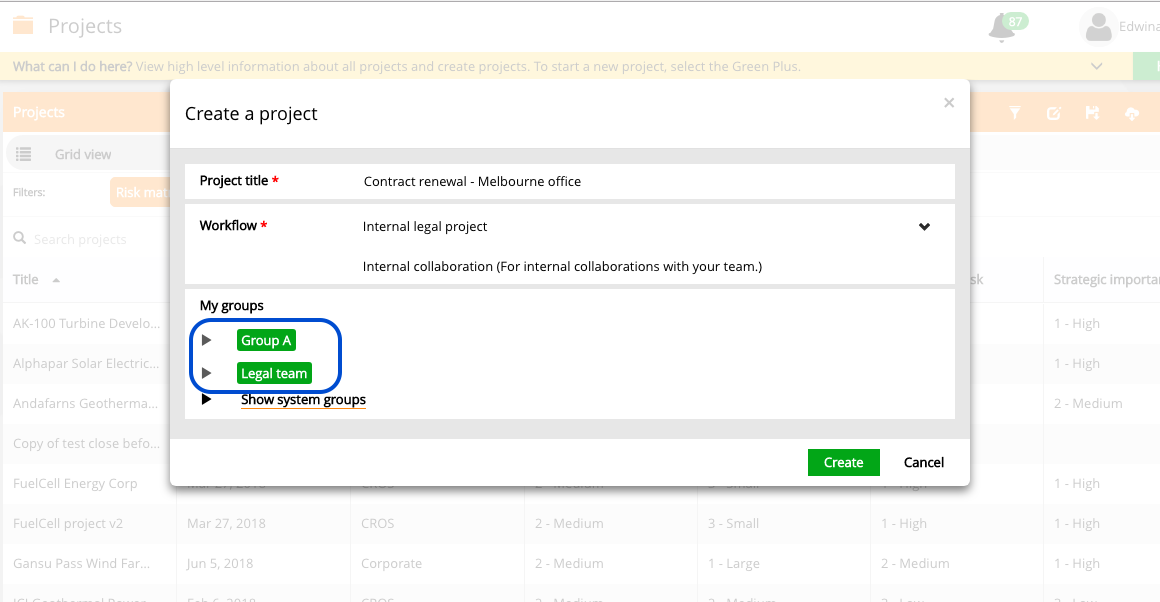The screenshot displays a project management application with an open dialog box positioned centrally on the page. At the top right corner, the word "Projects" is written in gray. The central pop-up dialog, bordered and accented with a slight shadow to suggest depth, bears the title "Create a Project" at the top, with a close icon ("X") positioned to its right.

The interface within the pop-up is organized into several sections. First, a labeled field "Project Title" appears with a text input box adjacent to it on the right. Beneath it, the label "Workflow" is displayed, followed by a dropdown box for selection purposes.

Further down, under the "My Groups" section, are two tags: "Group A" and "Legal Team," each encapsulated in green boxes. Notably, "Group A" is highlighted with a blue outline, indicating that it is currently active or selected. Adjacent to this, the "Show System Groups" label features a hyperlink styled as a link tree.

At the bottom right of the dialog, two action buttons are present — a green "Create" button and a white "Cancel" button, providing options to either finalize or discard the new project setup.

Partially visible behind the semi-transparent dialog is a dimmed view of the application's main interface, which appears to contain list-based project details reminiscent of an Excel sheet. To the left of the shadowed background is a navigation pane that is not fully visible in the screenshot.